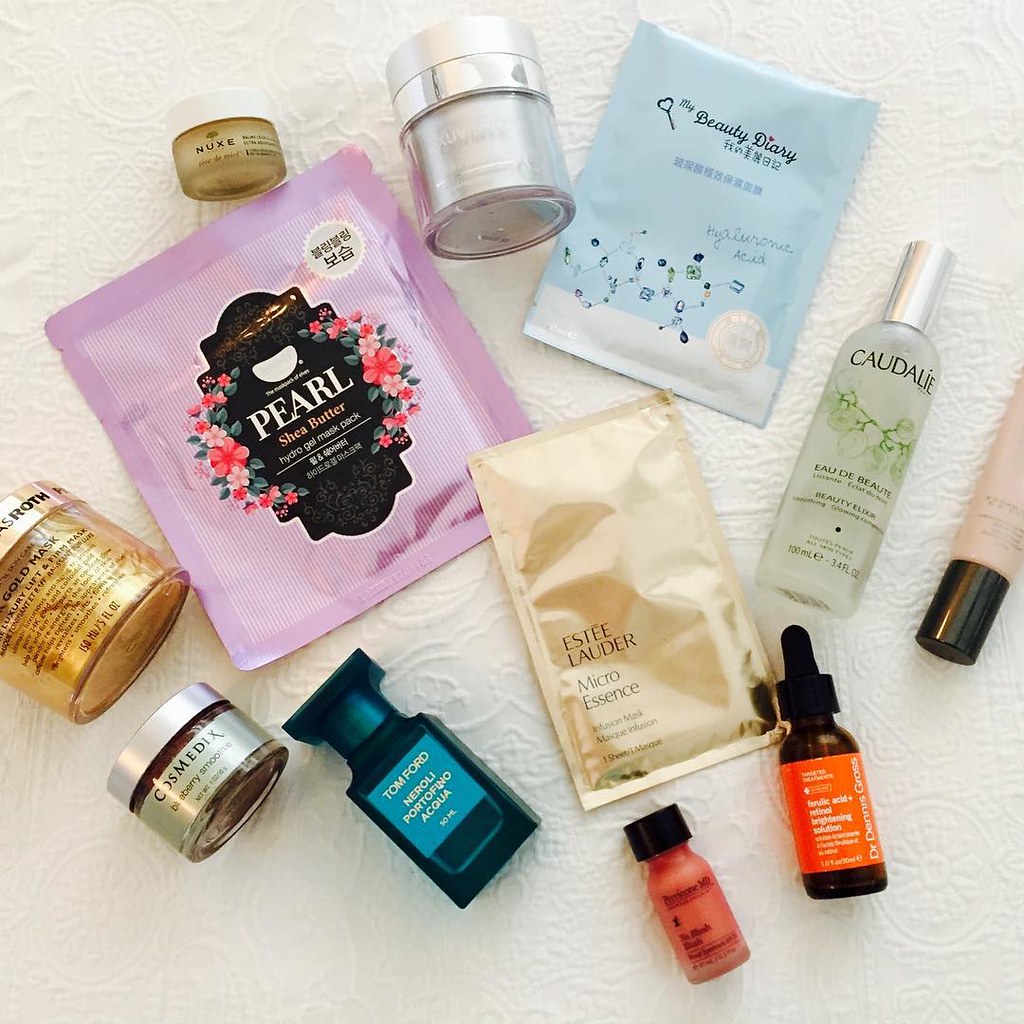The image showcases an assortment of beauty products meticulously arranged on a cloth-like surface. These items include several small bottles of gels and masks, each with unique branding and purposes. Notably, there's a prominent gold mask, albeit with the front label facing down, identified as the "Gold Max Luxury Lifting Mask."

Adjacent to it is a packet labeled "Pearl Shea Butter Hydrogel Mask Pack." Among the collection is a small product from the brand "NUXE," housed in a white bottle with an indeterminate silvery label. Also present is a packet from "My Beauty Diary," featuring Chinese text and mentioning "Hydraluronic Acid."

A bottle to the right is labeled "Beauty Elixir." There's also a small, nondescript bottle, the details of which are unreadable. Partially visible from the image's edge is a gold packet bearing the name "Estée Lauder Micro Essence."

Additionally, a dropper bottle from "Dr. Dennis Gross" claims to contain something related to acid and is described as an "Internal Initial Brightening Solution." Another small pink bottle with a red cap is present, although its label remains unclear. Finally, to the left, a distinctive blue bottle stands out, branded as "Tom Ford Neroli Portofino Aqua."

This variety of high-end beauty products suggests a focus on skincare and luxury, catering to various treatment needs.